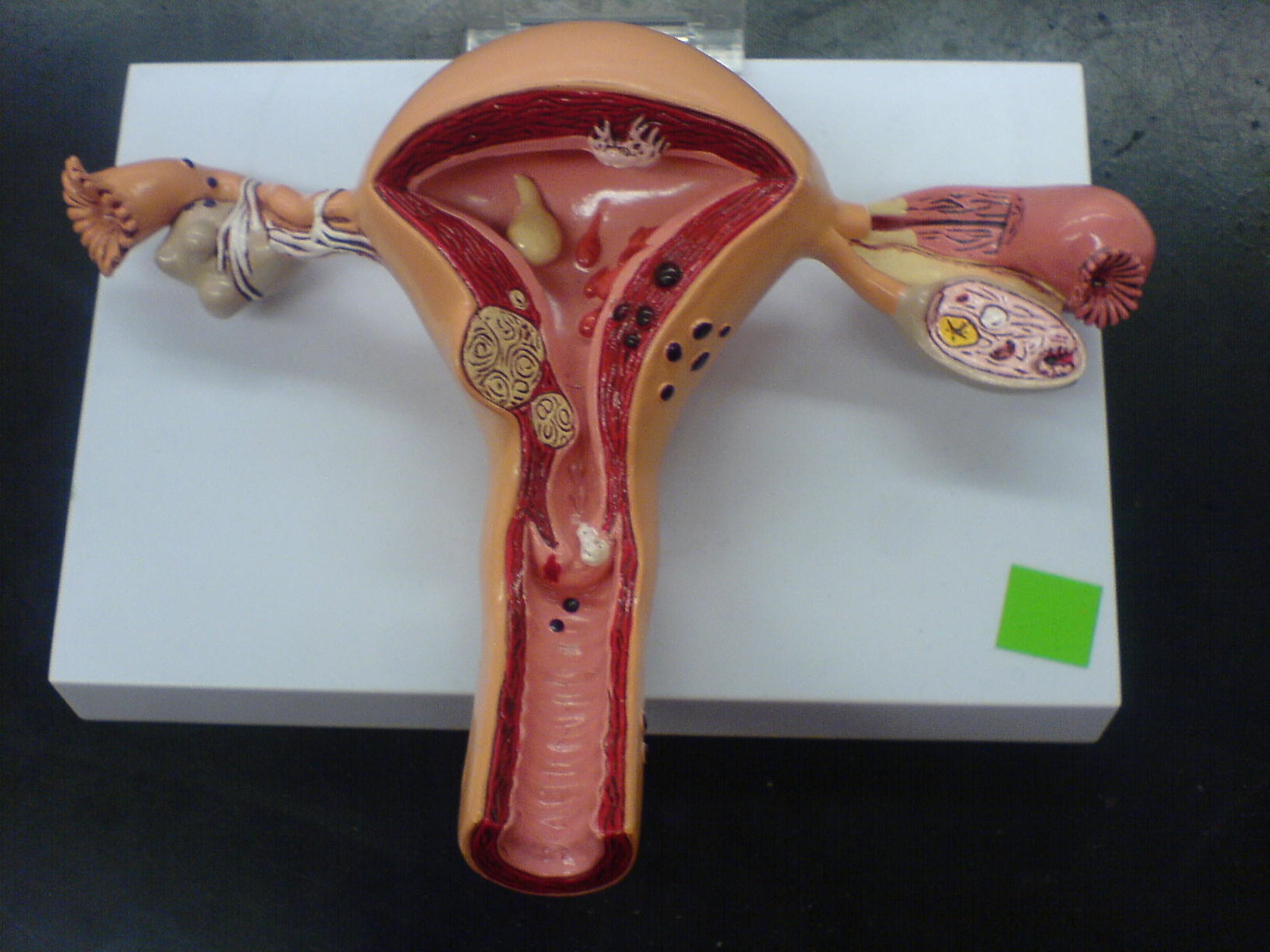This is a detailed image of a plastic model depicting a woman’s reproductive system, showcasing ovaries, fallopian tubes, and other internal structures. The model is color-coded with pink in the central areas, red outlining, and a beige flesh color on the outer parts. There are additional variations in color, including orange, red, and even blue dots. Small black specks can be seen, with two located inside and several on the outer sections, including four on the red parts. The entirety of the model is mounted on a white rectangular plastic block, and features a green square in the bottom right corner. The backdrop appears to include gray and blue hues, possibly of a wall or ceiling.